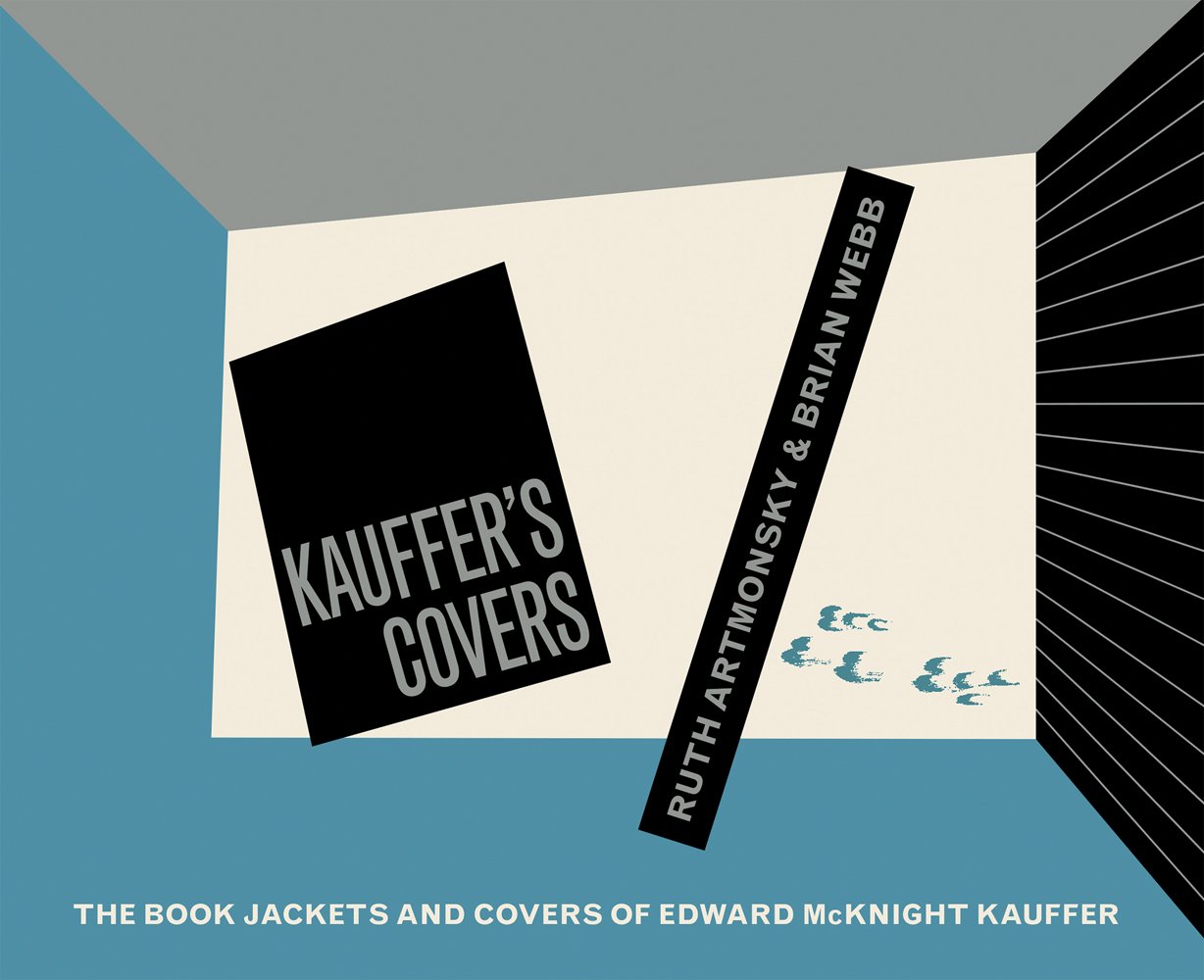The image is a meticulously designed digital poster with a 3D effect, creating the illusion of a small room. The ceiling is gray, the right side wall is black with white horizontal lines, and the floor and the left side wall are blue. The central wall is tinged with a tannish white background. Prominently placed in the center of the image is a black square tilted slightly to the left, bearing the title "Coffers Covers" in white text. Below the black square, the tagline "The book jackets and covers of Edward McKnight Coffer" is displayed in white letters. On the right side of the central wall, a vertical black rectangle features the names "Ruth Artmonski and Brian Webb" in gray text. The bottom right of the image is adorned with small, blue wave-like designs adding an intriguing visual element to the overall composition.